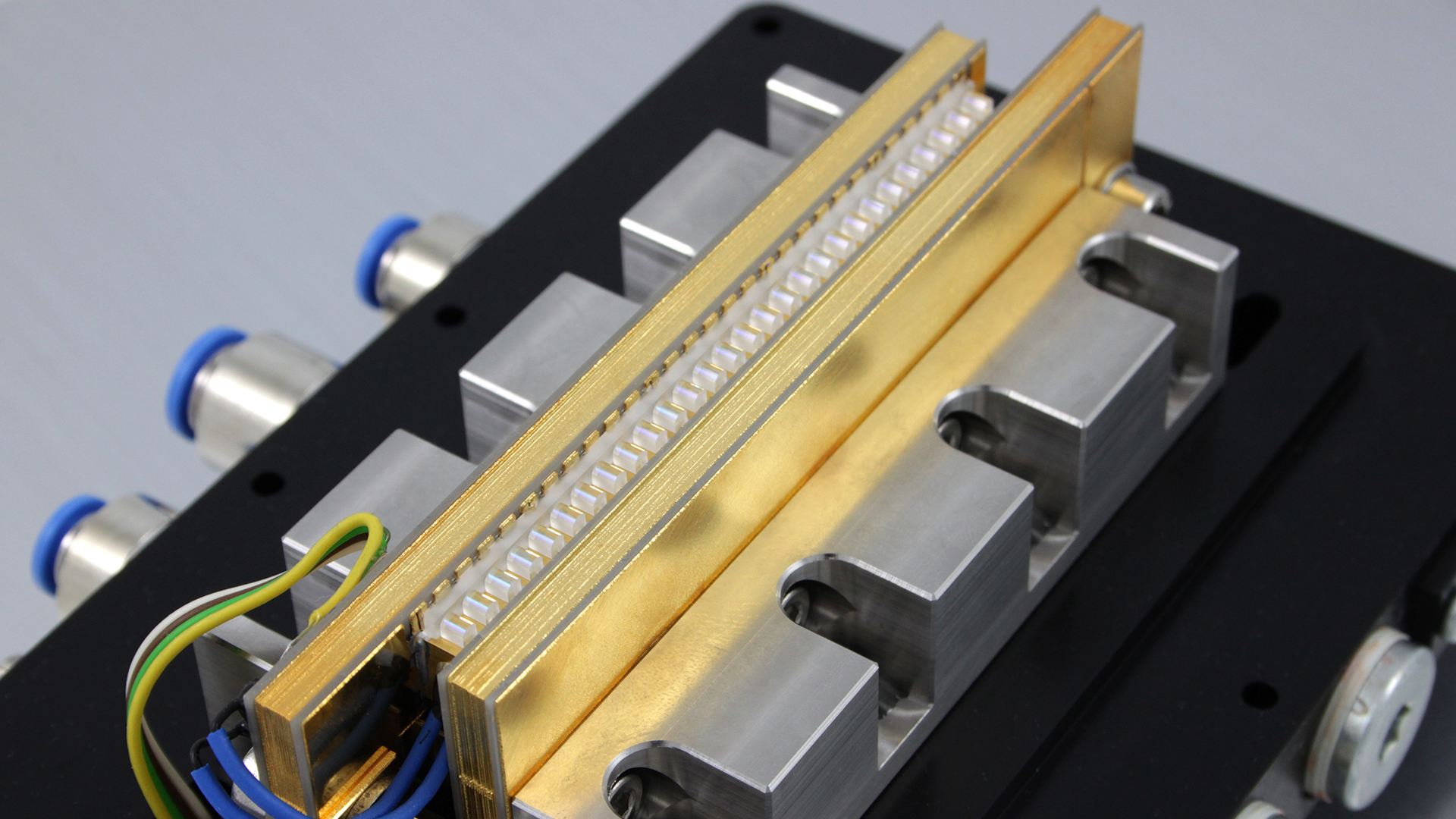The image displays an angled partial view of a black electronic device, set against a plain gray background, positioned diagonally from the bottom left to the upper right. On the left side, there are three protruding silver cylinders, each topped with blue buttons. Inside the uncovered black box, three rectangular structures are visible, revealing the inner workings of the buttons. A prominent feature in the middle is a gold component resembling a lopsided harmonica or a stack of pressed-together books, separated by white teeth-like pieces. The bottom left corner of the device houses an intricate bundle of wires, including yellow, green, red, blue, and white strands. A large screw is evident at the bottom right corner, likely part of the button mechanism from the opposite side. The setup suggests a mechanically complex and possibly electronic apparatus, with coaxial plug-ins and other components contributing to its functionality.